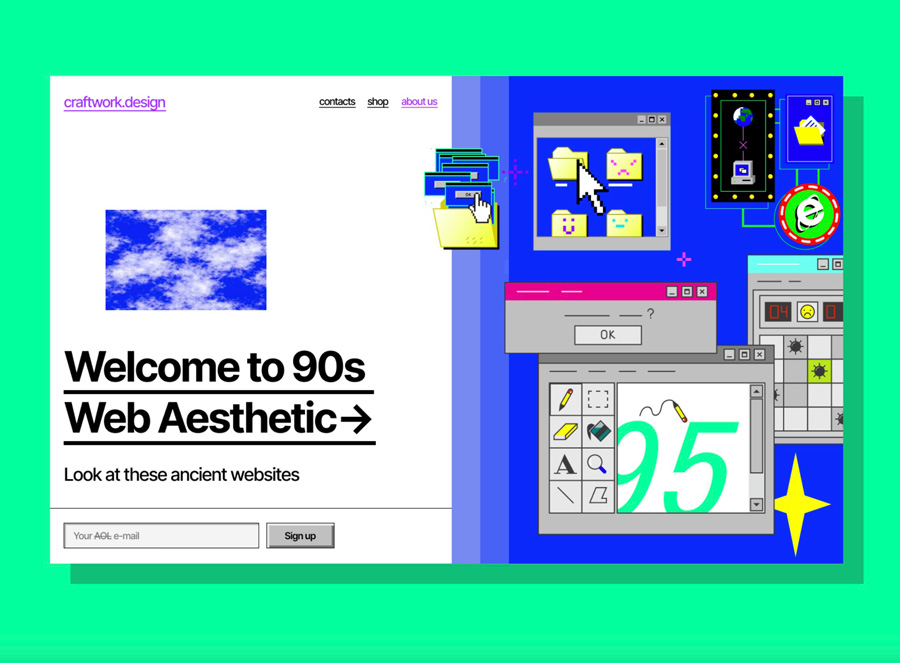The webpage for the company Craftwork.Design embraces a nostalgic 90s web aesthetic, prominently featuring a detailed retro design. At the top left, the Craftwork.Design logo is printed in purple, accompanied by a lime green frame that borders the entire page. The left side of the webpage has a white background, with a small image of a blue sky with white clouds beneath the logo. Below this image, the text "Welcome to the 90s Web Aesthetic" is boldly displayed in black and underlined, followed by "Look at these ancient websites."

The right side of the webpage showcases a blue background with a variety of 90s-inspired graphical elements. These include a computer monitor with lively yellow folder logos, reminiscent of early Windows interfaces, and a pop-up box with the word "OK" displayed in a pink-bordered rectangle. Scattered across this section are icons that harken back to classic 90s software and games such as Minesweeper and Paint, along with pixelated mouse pointers and the old Internet Explorer logo, further enhancing the retro feel of the design. Hyperlinks such as "Contact Shop" and "About Us" are also present, blending into the nostalgic theme of this creatively crafted advertisement.